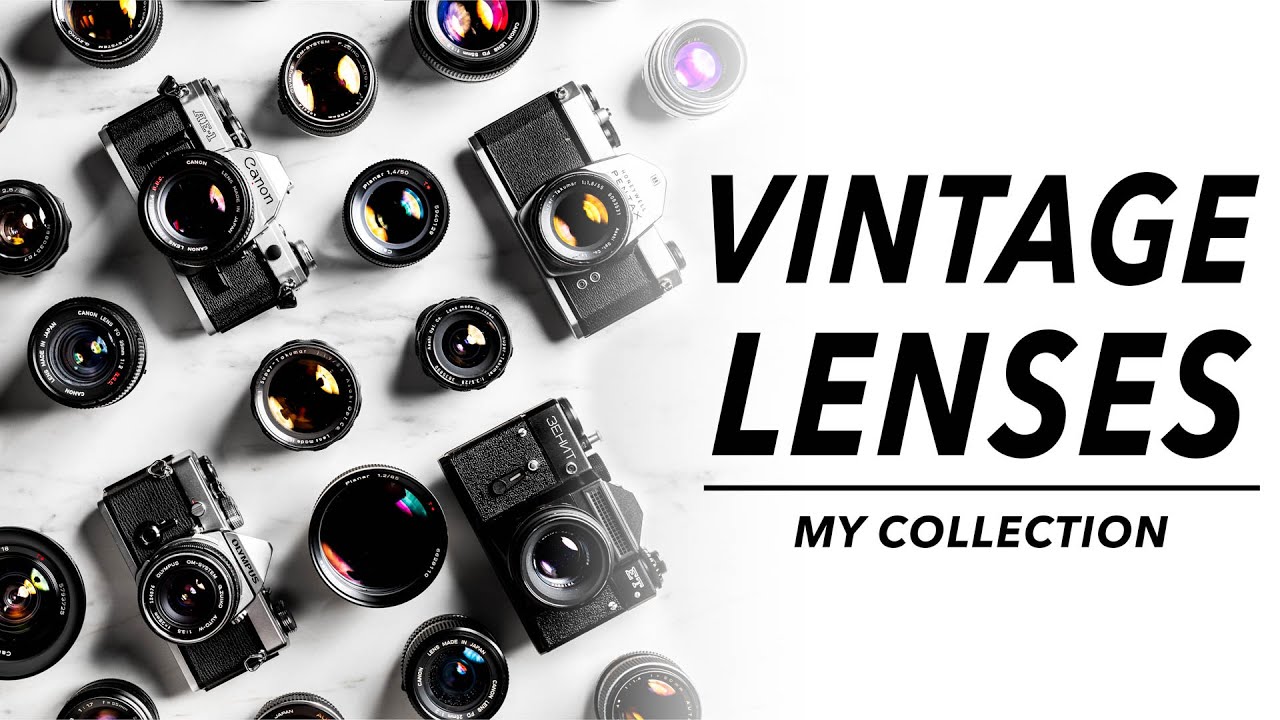The image appears to be a modern advertisement showcasing a collection of vintage lenses and cameras. The background is white with some gray streaks. On the right side of the image, in black text, it reads "Vintage Lenses," followed by a line and then "My Collection" in smaller letters. The left side of the image features four vintage film cameras - a Canon, an Olympus, a Pentax, and another identifiable by the label "3EH Backward NT." These cameras are laid out diagonally from left to right, with two of them having a silver top portion. Surrounding the cameras are numerous black lenses, approximately 12 to 13, all facing upwards, reflecting various colors like yellow, purple, red, blue, and pink due to the lighting. Each lens has words around its edge and is catching light that projects shadows towards the bottom left of the picture. The overall style of the image suggests it could be used as a thumbnail for a YouTube video, Pinterest, Instagram, or another social media platform, emphasizing the allure of vintage photography equipment.